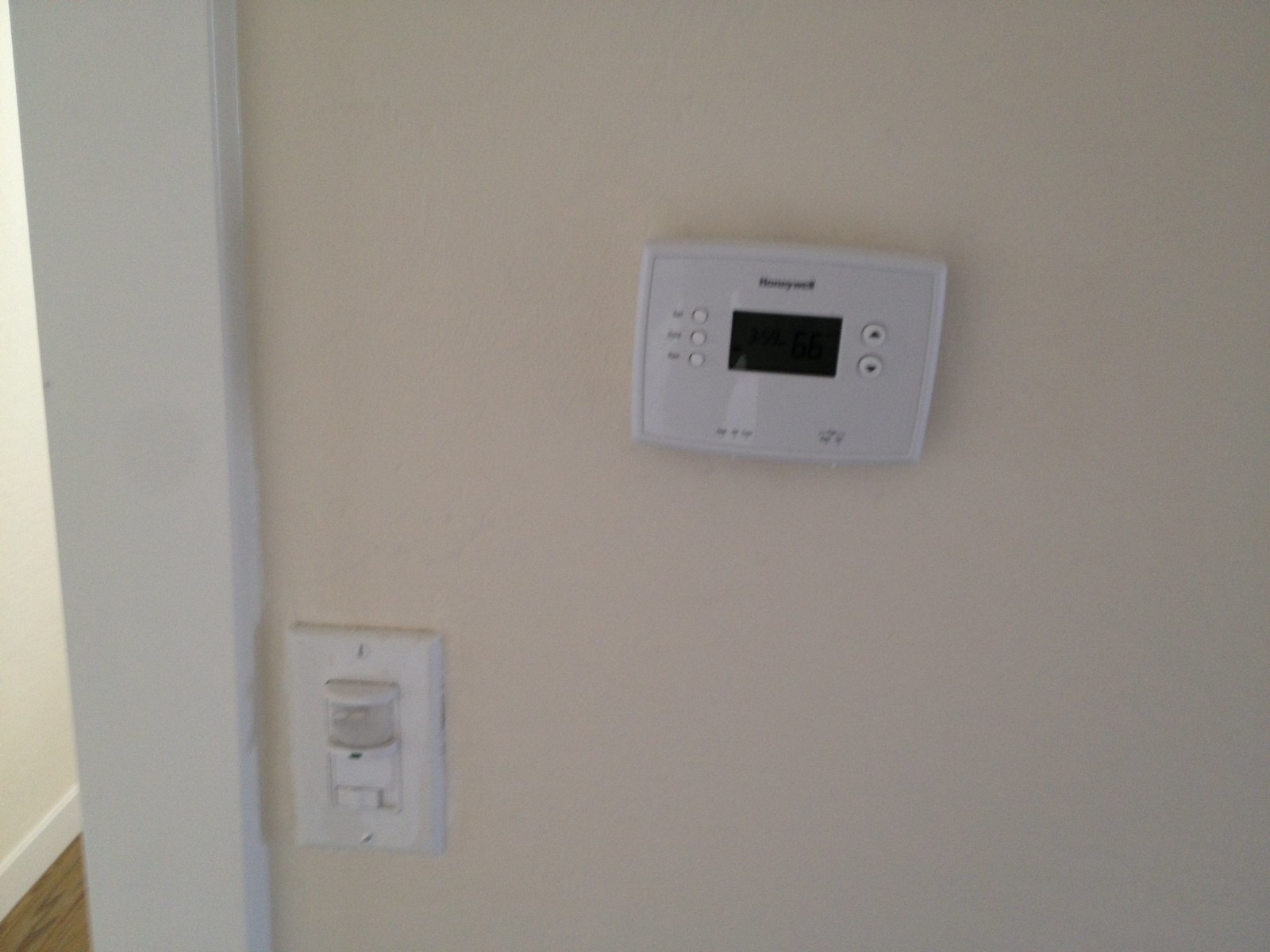The photograph captures a section of a tan-colored wall featuring a Honeywell thermostat and a light switch. On the bottom left edge of the image, a sliver of flooring is visible, suggesting that the wall ends in a hallway. Adjacent to the hallway, a white baseboard outlines what appears to be a doorway. Positioned in the lower middle portion of the wall, next to the white baseboard, is a standard light switch.

The centerpiece of the photo, the Honeywell thermostat, is mounted higher up on the wall. Although the display is difficult to read, it is prominently located in the middle of the device. To the left of the display are three round buttons, their functions unspecified. To the right of the display are two triangular buttons, one upright and one inverted, used for adjusting the temperature settings. Towards the bottom of the thermostat are various inscriptions likely indicating different modes, including 'off', 'heat', and 'cool', with additional settings on the lower-right corner. The scene captures the utilitarian elements of the wall within a residential or office space, highlighting the functionality and layout of these everyday components.